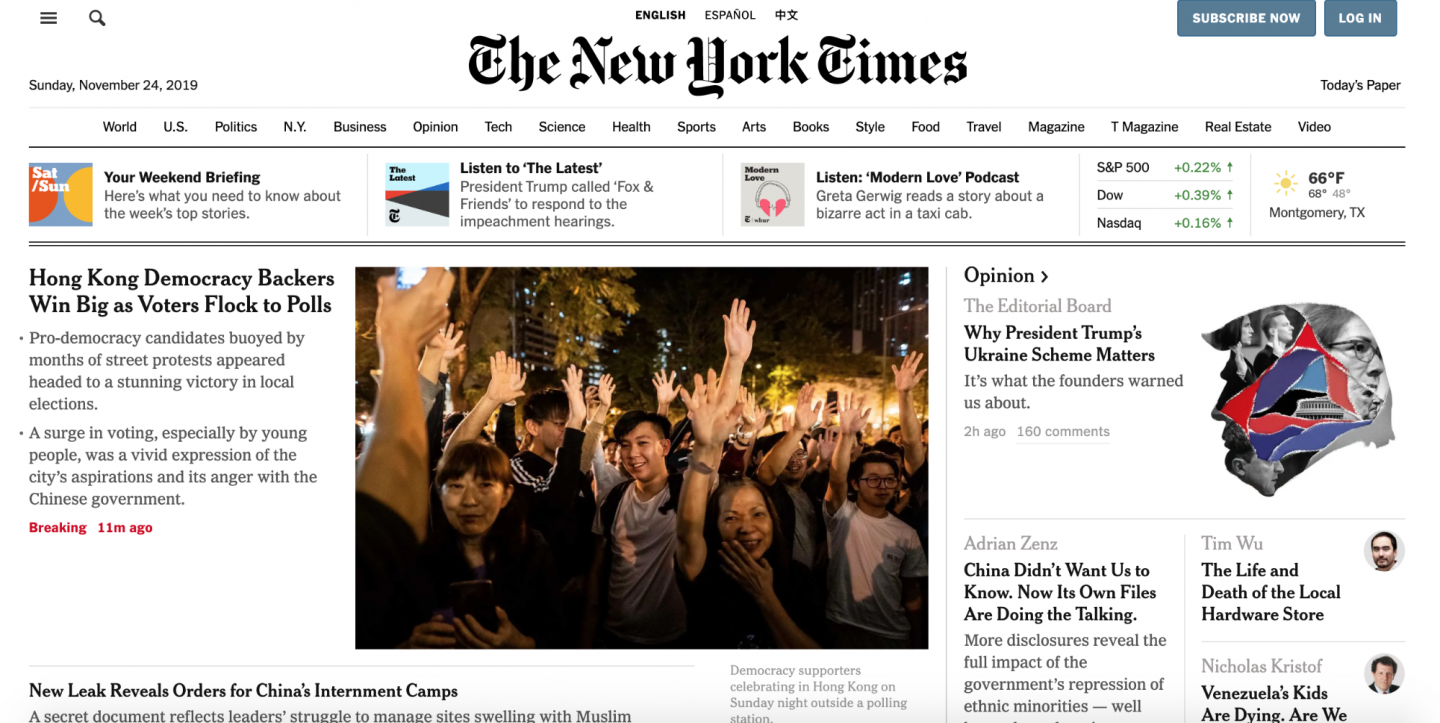The image depicts a screenshot of the New York Times website. The page has a white background with predominantly black text. In the upper left corner, there are two buttons: a menu list button and a search button. In the upper right corner, there are "Subscribe Now" and "Login" buttons. Centered at the top, the page offers language options in English, Español, and Japanese. 

The New York Times logo is prominently displayed in bold black letters in the center. Below the logo, a navigation bar contains tabs for various sections of the website, including World, U.S., Politics, N.Y., Business, Opinion, Tech, Science, Health, Sports, Arts, Books, Style, Food, Travel, Magazine, T Magazine, Real Estate, and Video.

Further down, the homepage features sections such as "Your Weekend Briefing" and "What You Need to Know About Upcoming Top Stories." There's a call-to-action for readers to "Listen to the Latest" and to tune into the "Modern Love" podcast. On the right side of the screen, there is a widget displaying stock information and weather updates.

The main body of the content includes articles, with one focusing on Hong Kong democracy, accompanied by relevant images. Additional article snippets and images are also visible on the right side of the page.